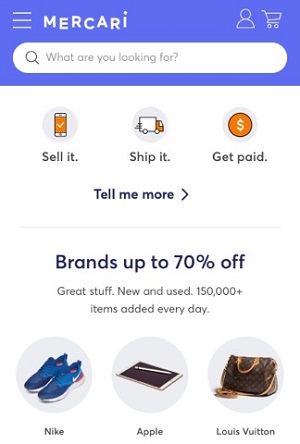This image is a detailed screenshot of the Mercari website homepage. At the top, there is a wide blue banner featuring a horizontal menu icon comprised of three lines in the upper left corner. Next to the menu icon is the Mercari logo, characterized by uneven lettering. On the right side of the banner, there are icons for the user's account and a shopping cart, both in white.

Beneath the banner, a white search bar is prominently displayed with a grey magnifying glass icon and placeholder text that reads, "What are you looking for?" Below the search bar are three actionable options: "Sell it" on the left, followed by "Ship it" with an icon of a truck in orange and white, and "Get paid" with a circle icon featuring a white dollar sign. Below these options is a "Tell me more" link in bold text with an arrow pointing to the right.

Further down, the banner showcases a promotional message in bold text, "Brands up to 70% off," followed by a subtext in light grey, "Great stuff, new and used."